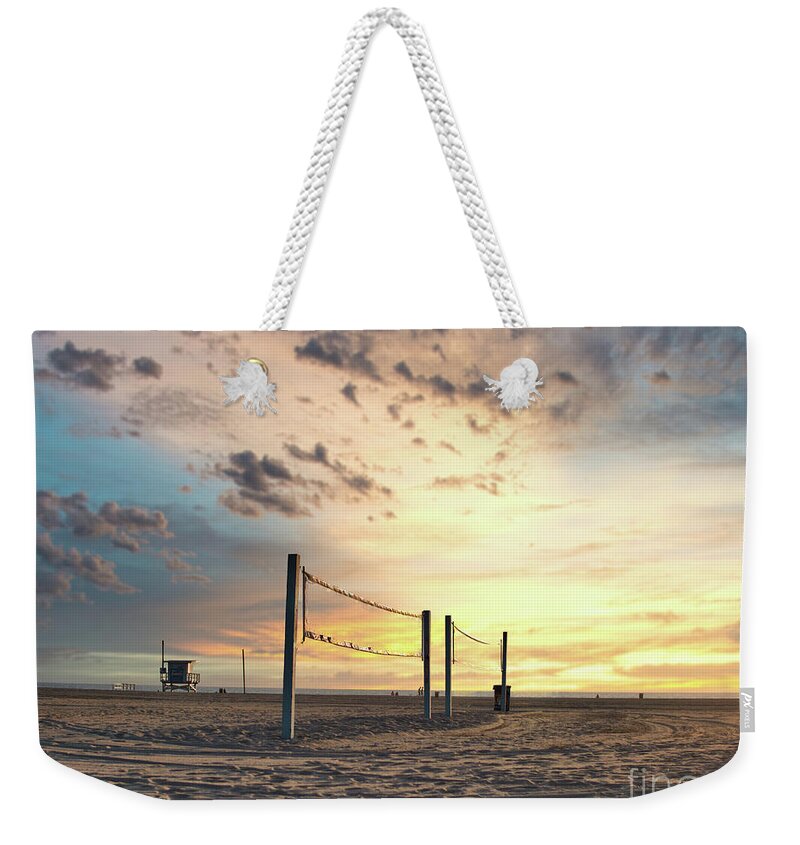The image is a detailed color photograph of a tote-style bag. The bag, lying flat with its front side facing up, features a rope handle threaded through two grommets at the top, with its ends frayed. The handle is stretched into a triangle shape. A tag reading "PX" and another unreadable word hangs off the right side of the bag. The entire front of the bag is printed with a vivid beach scene depicting a volleyball field. The sandy field is adorned with two volleyball nets arranged side by side, and in the distant background, an ocean can be seen. The serene sky above ranges in beautiful hues of blue, purple, yellow, and orange, giving the impression of a sunset. Fluffy clouds scattered throughout add to the tranquil atmosphere. Additionally, a lifeguard tower is positioned to the left within the scene, completing the picturesque beach setting.